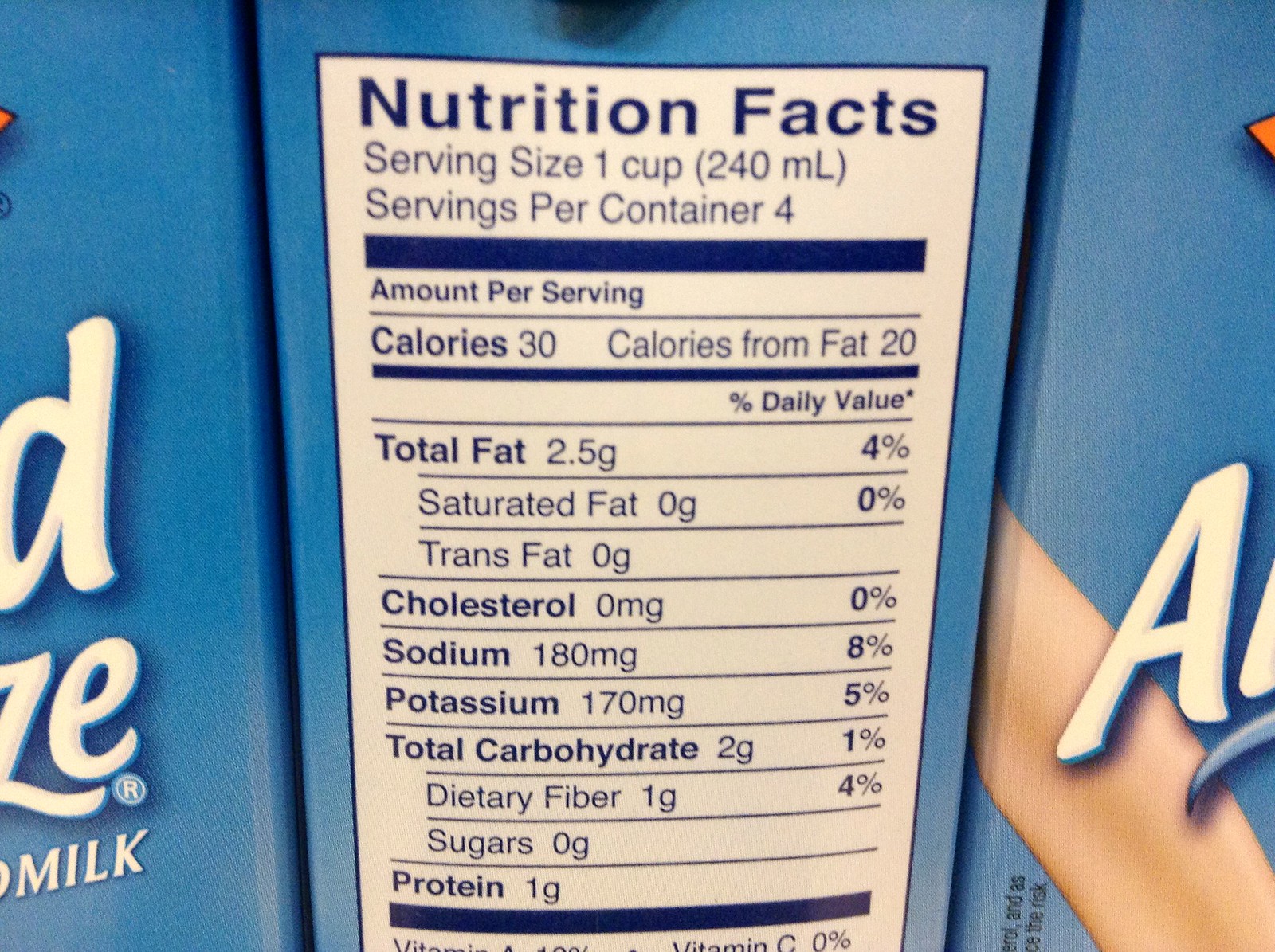The image depicts the detailed back label of an almond milk container. Prominently featured in the center of the image are the nutrition facts, which are laid out clearly. At the top of the label, the serving size is indicated as one cup, with approximately four servings per container. Each serving contains 30 calories, 20 of which are from fat. The total fat content is 2.5 grams, constituting 4% of the daily value. The cholesterol content is zero. Sodium is listed at 180 milligrams, and potassium at 170 milligrams. The total carbohydrate content is 2 grams, accompanied by 1 gram of protein. Additionally, the partially visible words to the left and right suggest branding elements, with the word 'milk' discernible in smaller font beneath these fragments. The detail in the description emphasizes the nutritional content as the focal point of the image.